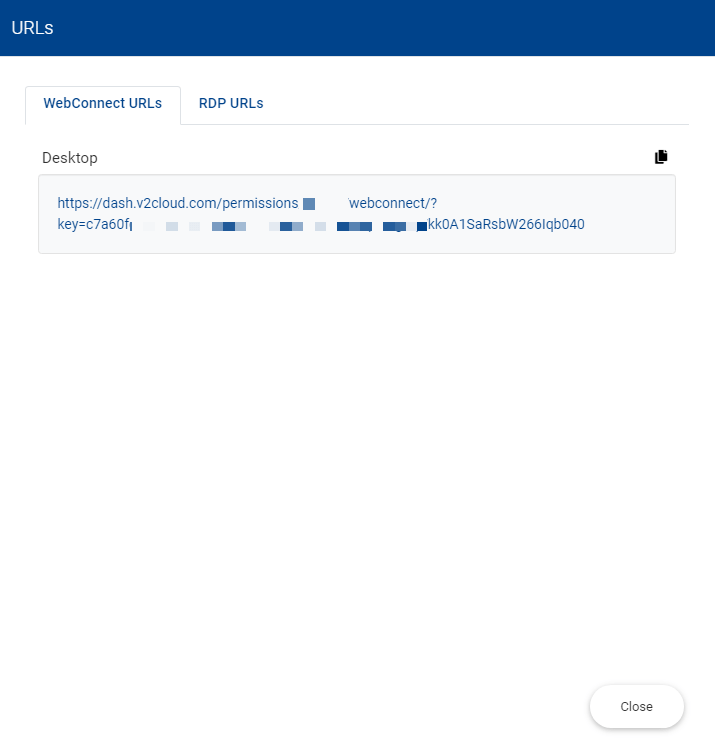The screenshot features a white background with a dark blue horizontal rectangle spanning across the top. On the left side of this rectangle, centered vertically, there is white text displaying the URL in lowercase.

Below this, there are two tabs slightly indented:
1. The first tab contains blue text that reads "WebConnect." A light gray line runs vertically to the left of this tab and horizontally to the right.
2. To the right of the first tab, there is blue text reading "RDP."

Approximately two lines below these tabs, the word "Desktop" appears in gray text.

On the right side of the image, there is a page icon. Below this icon is a light blue rectangle outlined with a light gray line. To the right of this rectangle, blue text displays the URL "https://dash.v2cloud.com/permissions."

Further to the right, approximately four spaces after the URL, there is a blue square followed by blue text reading "WebConnect/?"

The next line down contains blue text: "key=C7A60FI." Further to the right, there are several horizontal rectangles filled with varying shades of blue squares inside them. To the right of these rectangles, small blue letters spell out "KKDA1SARSBW266LQB040."